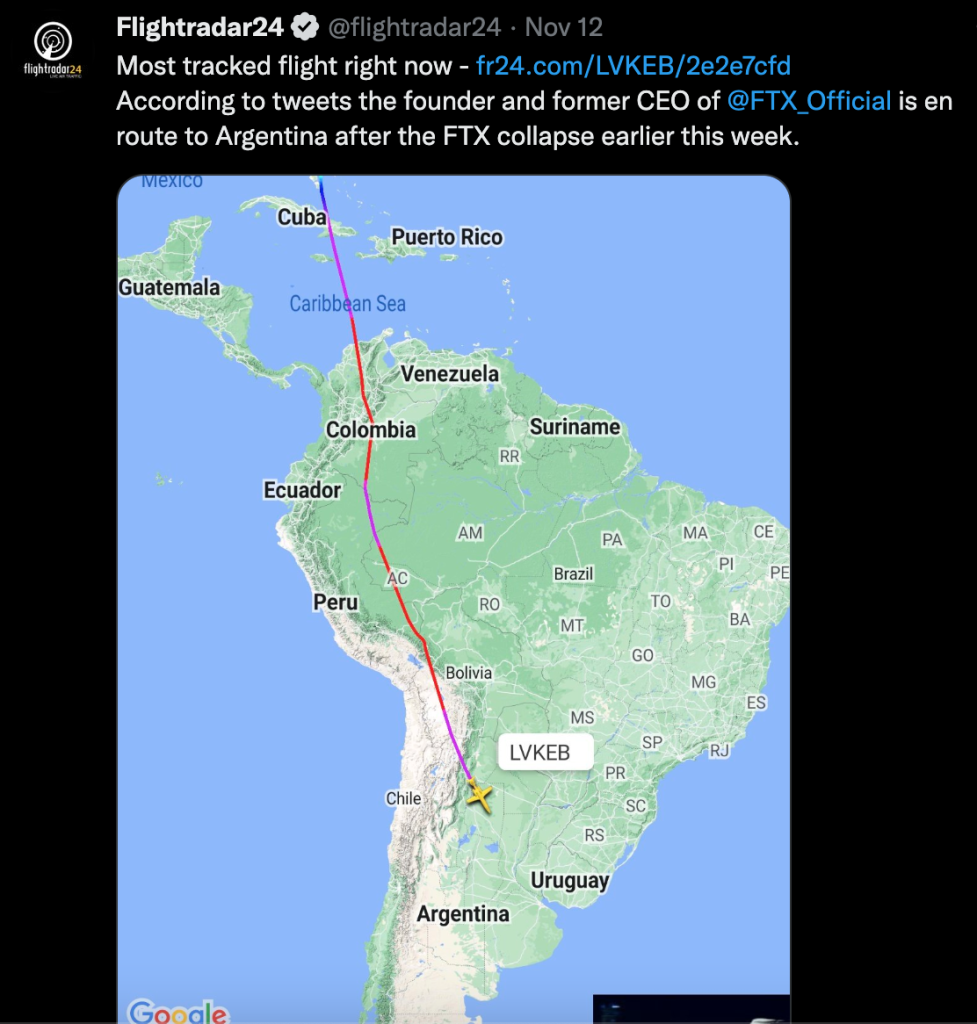This image is a social media post from Flight Radar 24, showcasing their sleek black background with predominantly white text and some blue hyperlinks. At the top, the post prominently features, in bold white letters, "Flight Radar 24," accompanied by a white ribbon and black checkmark, suggesting verification. Adjacent to this, it reads "@FlightRadar24," followed by the date "November 12th" with no specified year. On the upper left corner of the post is Flight Radar 24's logo, which consists of a radar icon.

The main content of the post highlights the "most tracked flight right now" with a clickable blue link: "FR24.com/LBKEB/2E2E7CFD." The text elaborates that, according to tweets, the founder and former CEO of "@FTX_official," is reportedly en route to Argentina following the recent collapse of FTX.

Beneath the textual post, there is a detailed map image depicting the continent of South America along with parts of Central America, Puerto Rico, and Cuba. The map includes labels such as "Mexico" in the Gulf of Mexico and "Caribbean Sea" with various cities marked. A multicolored flight path is superimposed on the map, culminating in a yellow airplane icon, ostensibly indicating the current location of the tracked flight mentioned in the tweet.